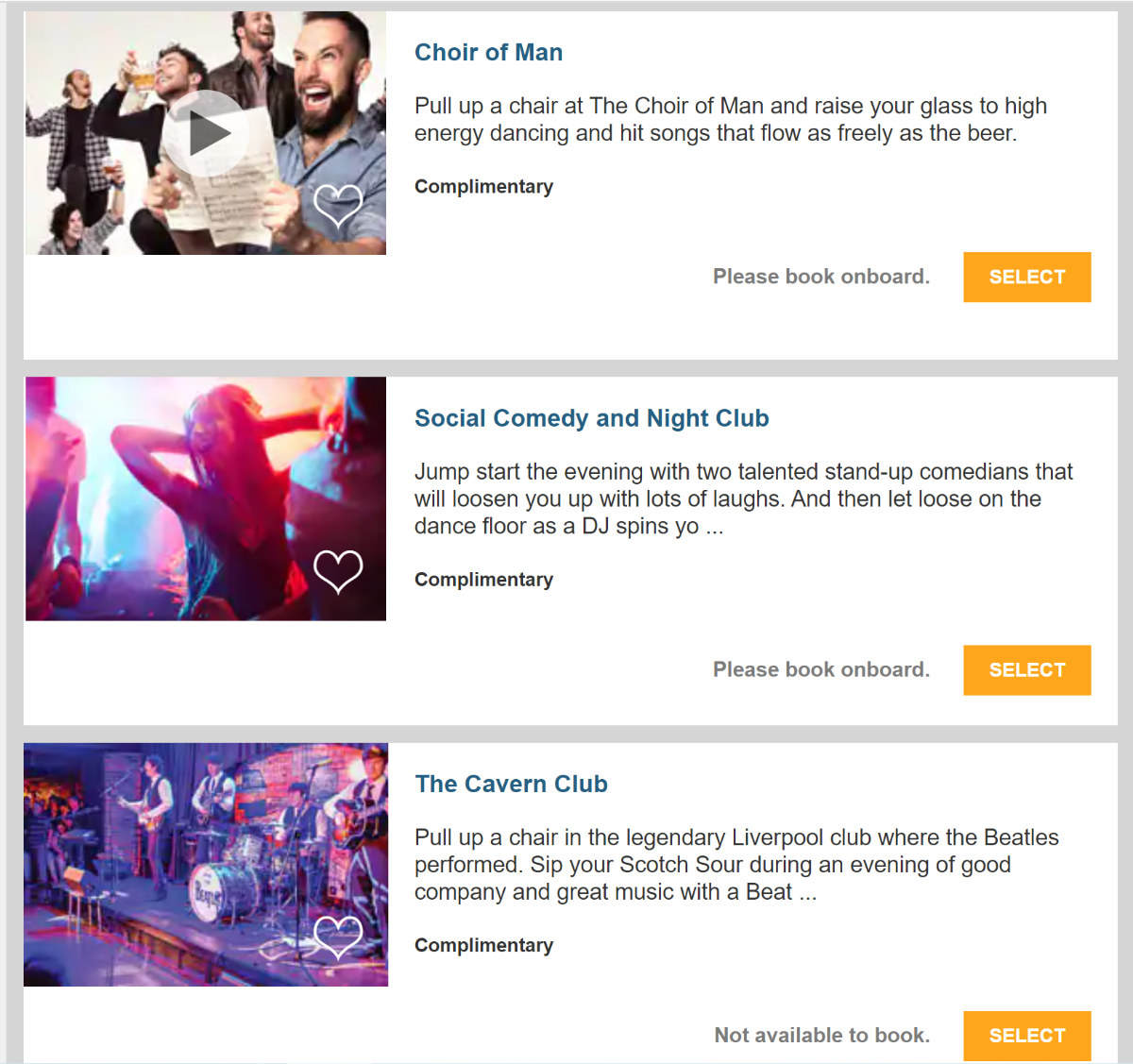### Detailed Caption for the Series of Images:

This series of three images showcases different entertainment offerings, each framed with a thin gray border and set against a white background. Each image features a blue title with about two sentences of black text detailing the event.

1. **Image Title: Choir of Man**
   - **Visual Description**: This image features a group of men, most of whom have dark hair. One man in a blue shirt is holding what appears to be a piece of sheet music and is laughing hysterically. Another man lifts a glass of beer in a jubilant toast, while another, dressed in plaid, similarly has a drink in hand.
   - **Text Description**: "Pull up a chair at the Choir of Man and raise your glass to high-energy dancing and hit songs that flow as freely as the beer. Complimentary." There's a white heart symbol and a note that says, "Please book on board." A gold and white box below reads "Select."

2. **Image Title: Social Comedy and Nightclub**
   - **Visual Description**: The image depicts a woman in a club setting, her arms raised behind her head, laughing. She has long hair and is wearing a black shirt. The background is lit with pink and blue neon lights, creating a vibrant atmosphere.
   - **Text Description**: "Jumpstart the evening with two talented stand-up comedians that will loosen you up with lots of laughs, then let loose on the dance floor as a DJ spins." The description cuts off at this point. It also mentions that this event is complimentary with a note "Please book on board." Below is a gold and white box labeled "Select."

3. **Image Title: The Cavern Club**
   - **Visual Description**: This image likely features a Beatles tribute band, with dark-haired men playing instruments on a stage. In the audience, a few people can be seen enjoying the performance.
   - **Text Description**: "Pull up a chair in the legendary Liverpool club where the Beatles performed. Sip your scotch sour during an evening of good company and great music with a beat." This text also cuts off mid-sentence. It’s noted as complimentary, but not available to book. There is a gold and white box that says "Select."

Each of these images presents a different vibrant experience, emphasizing high-energy performances, laughter, and memorable music, ultimately encouraging viewers to join these complimentary onboard activities.